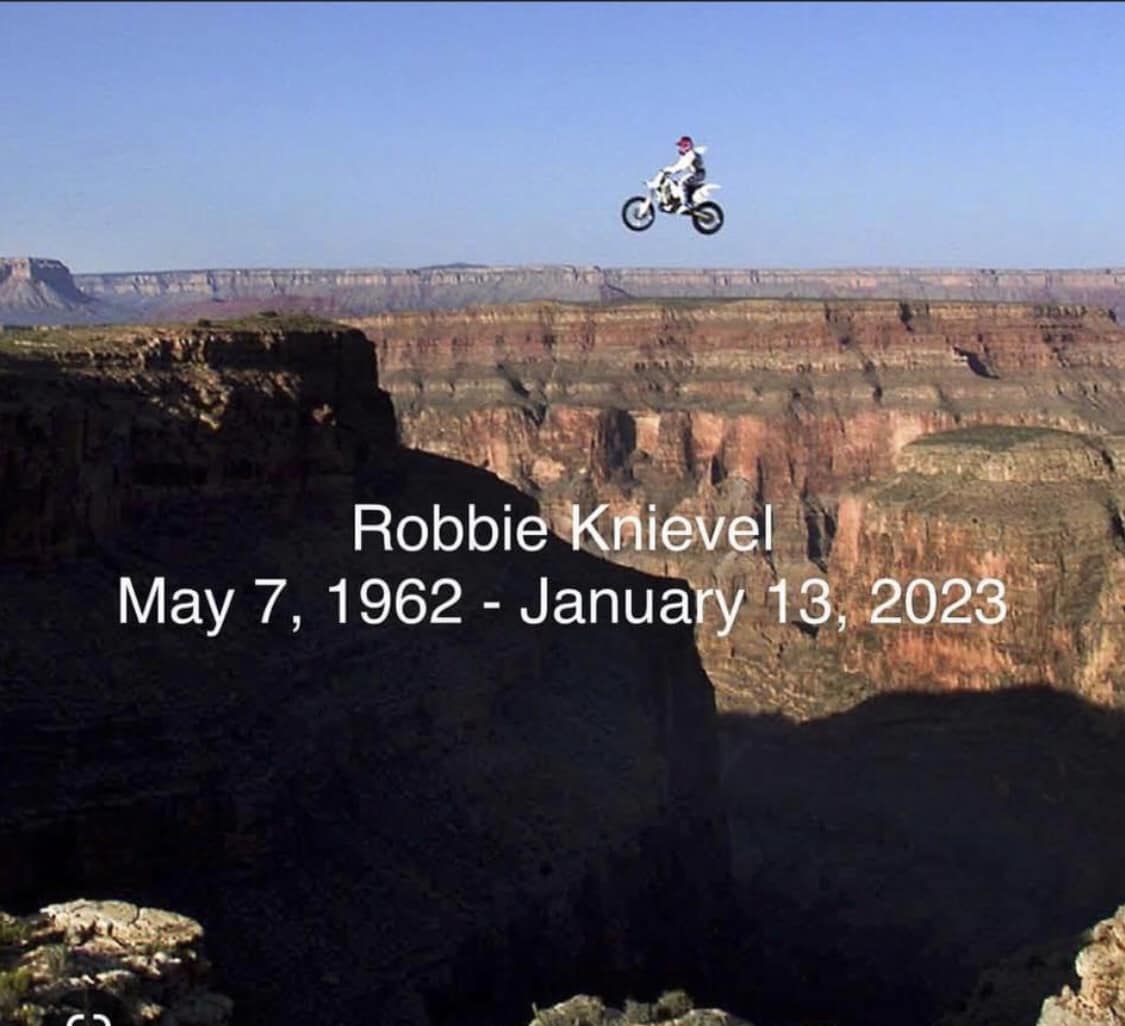The image captures a heart-stopping moment of Robbie Knievel airborne on his motorcycle, mid-stunt over a vast canyon with a dizzying drop-off. The blue sky serves as a pristine backdrop, devoid of clouds, highlighting the dramatic leap. Below, the rugged terrain of the canyon with its rocky outcrops and distant hills is shadowed, intensifying the sense of depth and danger. Robbie, identifiable by his white suit and red helmet, pilots a white motorcycle adorned with black wheels. Centered in the image is a tribute in white text: "Robbie Knievel, May 7th, 1962 to January 13th, 2023," memorializing the legendary daredevil who recently passed away. The setting sun casts dark shadows at the bottom, emphasizing the perilous nature of the stunt, possibly reminiscent of the expansive canyons of Arizona, echoing the grandeur and risks reminiscent of the Knievel legacy.